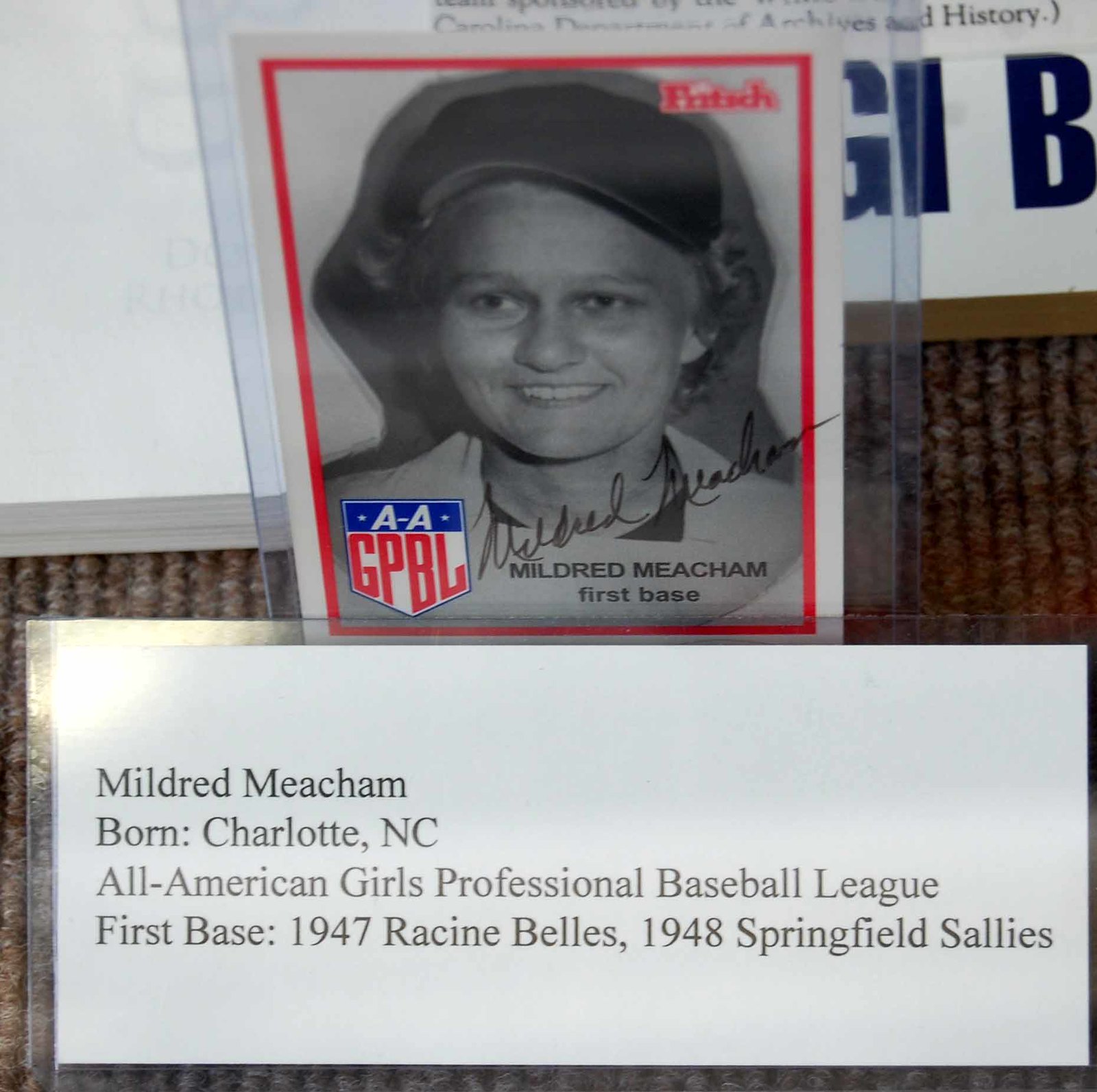The image features a black-and-white photograph of a smiling young Caucasian woman with light brown to dirty blonde short curly hair, wearing a baseball cap. She is showcased on a trading card that seems to be protected by a clear plastic cover. The card itself has a white background with a red inner border. Just above the woman’s shoulder, there's a signature scrawled diagonally and ascending across the base of her neck. To the left of her shoulder area, the card has a logo with white text "AA" on a blue background, and below it "GPBL" in red text on a white background, representing the All-American Girls Professional Baseball League. At the bottom of the card, her name, "Mildred Beauchamp," and her position, "First Base," are printed in black, all caps for the name and lowercase letters for the position. To the upper right, the card is marked with a small, somewhat blurry, shield logo starting with "F" and ending with "H" in red. The trading card is positioned against what appears to be a short-haired brown fabric, possibly a rug. Below the card, a white laminated strip of paper details her biography, stating: "Mildred Beauchamp, born Charlotte, NC, All-American Girls Professional Baseball League, First Base, 1947 Racine Bells, 1948 Springfield Sallies."